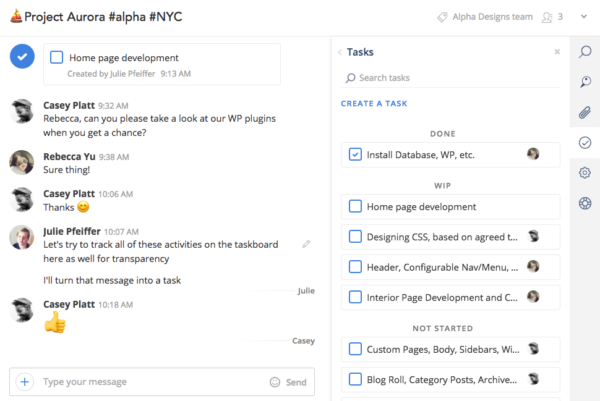**Caption:**

The image is from Project Aurora, tagged #Alpha and #NewYorkCity, featuring a web page in development. The top left showcases a blue circle with a white checkmark, indicating "Homepage Development." The page is bustling with activity: users are actively posting updates and collaborating. One user, Rebecca, is asked to review web page plugins, to which she promptly agrees. Another user suggests tracking all activities on a task board for transparency and converts the message into a task, receiving a thumbs-up in response.

On the right side, there's a detailed task list with categories: a search bar labeled "Create a Task," followed by statuses like "Done," "WIP" (Work in Progress), and tasks yet to be started. The sections include "Homepage Development," encompassing tasks like designing headers, interior pages, custom pages, body, and sidebars. Another section, "Blog Role," lists tasks related to posts and archives. Completed tasks are marked with a checkmark in their respective boxes.